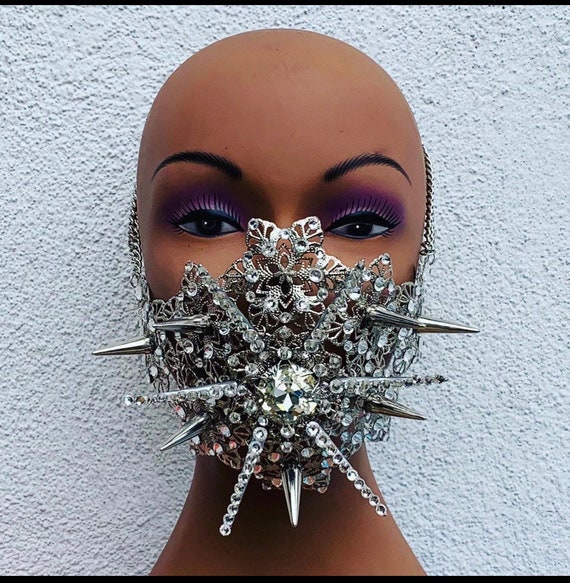The image is a highly detailed, computer-generated depiction of a bald woman standing against a textured, white, concrete-like wall. Her head, completely devoid of hair, features meticulously drawn black eyebrows and long, black eyelashes framing dark eyes accentuated by purple eyeshadow. The lower half of her face, starting just below her eyes and extending past her nose and mouth, is obscured by a striking metallic mask. This elaborate mask is encrusted with dazzling diamonds and various shiny jewels, and adorned with spikes that jut out prominently at several points — notably near the cheekbones, cheeks, bottom lip, and chin. Two chains extend upward on either side, appearing to secure the mask in place. The mask's design also includes intricate metallic elements and leaf motifs, blending spikes and gem-like adornments to create a dramatic, avant-garde effect.